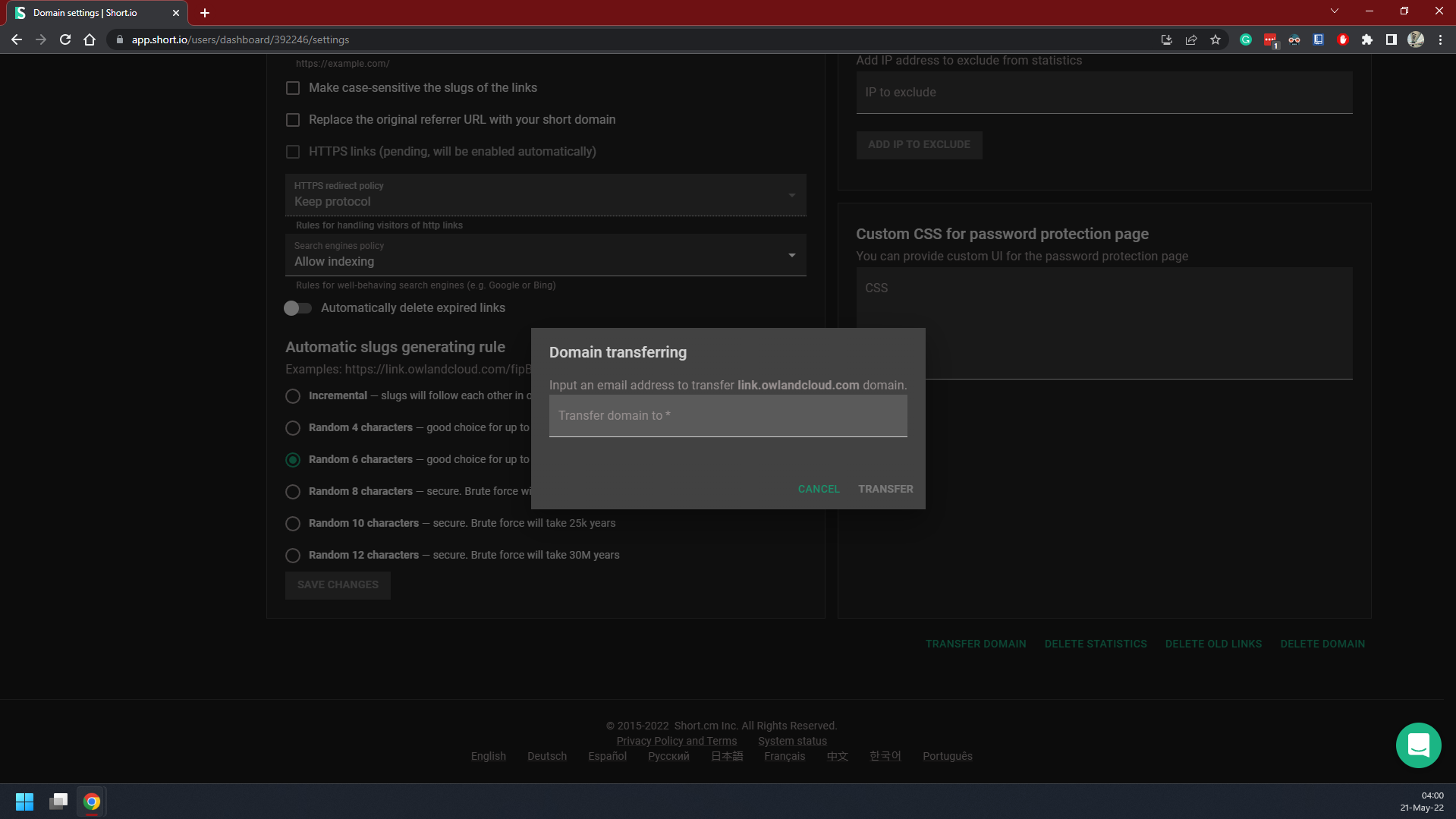The image captures a detailed view of a computer screen. The background is black with a prominent red border at the top. In the upper left-hand corner, various computer logos are displayed. Beneath this, there are several buttons enriching the interface. 

At the top of the screen, the website address is visible as "app.short.lio/users/dashboard/392246/settings." The central portion of the screen features white text against the dark background, organized into columns. The first column includes a link option labeled "Make Case Sensitive the slugs of the link." Adjacent to it is another instruction: "Replaces the original referrer URL with your short domain."

Further down the page, a gray box stands out with the title "Domain Transferring" in white text. Below this, it instructs, "Input an email address to transfer link.owlandcloud.com domain." The main action is centered in the middle with the text "Transfer domain to," accompanied by two buttons at the bottom labeled "Cancel" and "Transfer."

At the very bottom of the screen, centrally located, the text reads, "2015-2022 short.cm Inc. All rights reserved. Privacy Policy and Terms. System Status." Additionally, there is a list of different languages available, enhancing the accessibility of the interface.